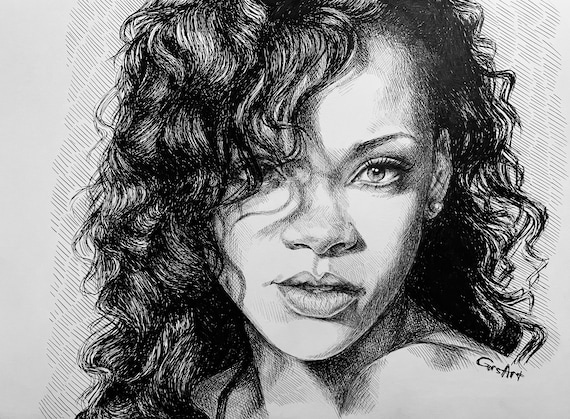The image is a detailed pencil drawing of the pop artist Rihanna, rendered in black and white. The portrait shows her staring directly at the viewer, with her wavy, dark hair parted to the side and cascading over her right eye and ear, leaving only the left side of her face fully visible. Her striking features include a broad nose, big lips, and blue eyes, although the black and white medium might affect the perception of her eye color. She is adorned with a small pearl stud earring in her left ear, and her hair extends behind her left shoulder. The background starts as a plain gray and transitions into horizontal diagonal lines, creating a shaded effect. An autograph, "GRS Art," is penned on her left shoulder, possibly indicating the artist. This headshot drawing focuses solely on her face and shoulder, with no clear indication of her clothing.